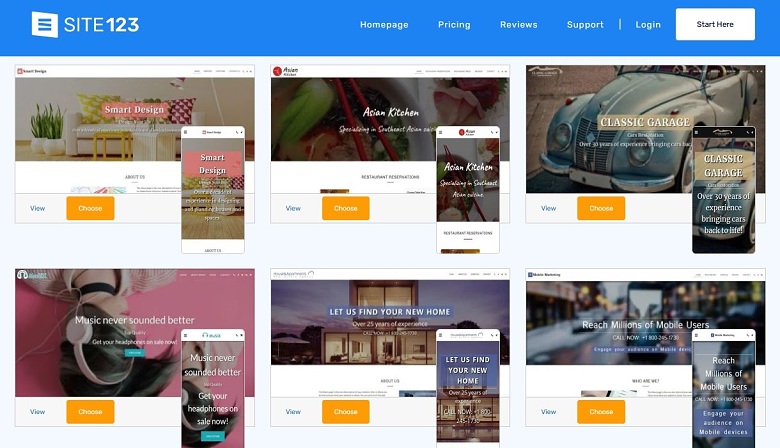Screenshot from the Site 123 website. In the upper left corner, the "Site 123" logo is prominently displayed. The top navigation bar is a blue horizontal rectangle featuring several tabs: "Homepage," "Pricing," "Reviews," "Support," and "Login." A white button labeled "Start Here" is also present.

Below the navigation bar, the layout consists of six images organized into three columns and two rows. Each image showcases design styles meant for creating personalized homepages or apps. 

In the top-left image, the template is branded "Smart Design," with a smartphone overlay on the right that displays the same "Smart Design" logo. This pattern of showing a desktop version and a mobile version side-by-side is consistent across all six templates.

Below each template, there are "View" and "Choose" buttons, allowing users to preview and select their preferred design. These templates appear to be pre-made designs for users looking to set up a website or app through Site 123, simplifying the creation process by offering a variety of customizable options.